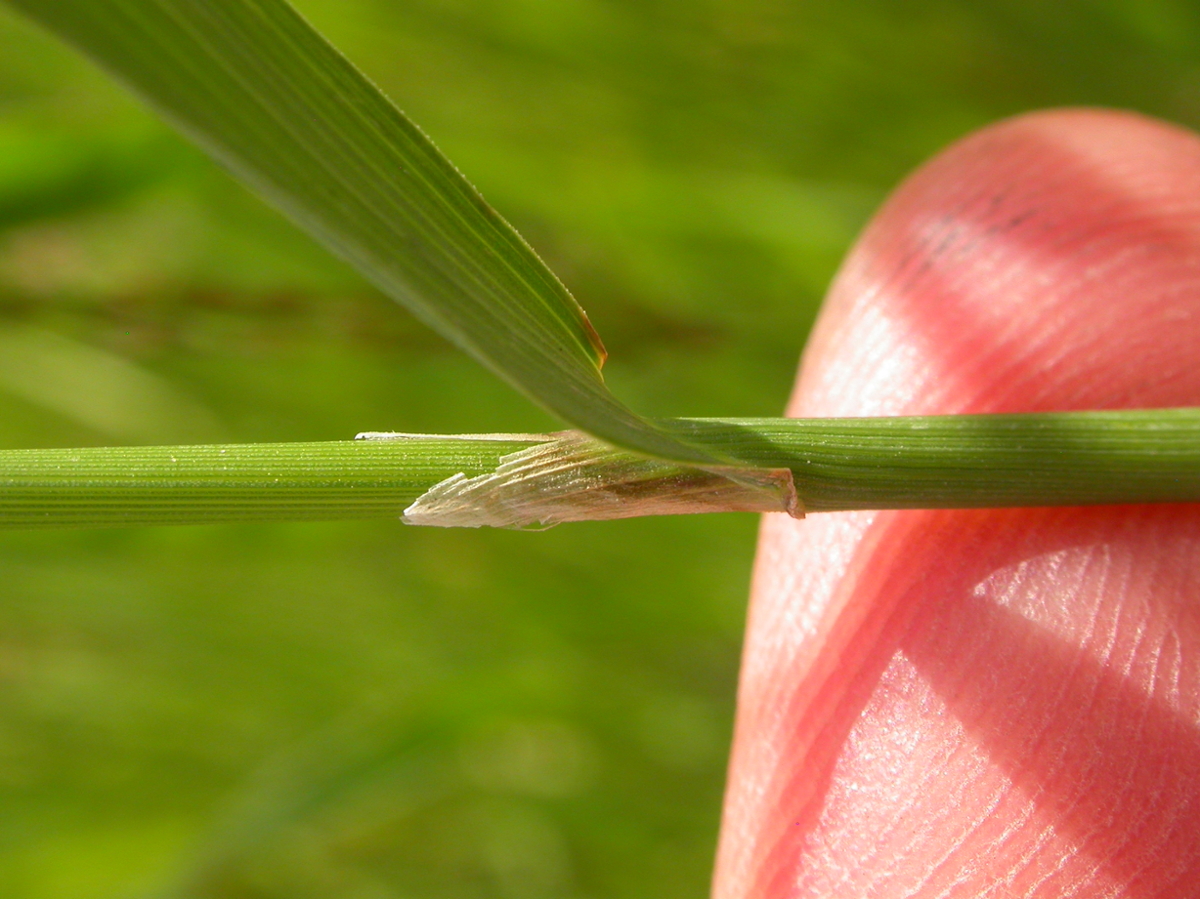The image is an extreme close-up of a pale pink human fingertip taking up most of the right side of the frame. The detailed ridges and lines of the fingerprints are clearly visible, as well as the subtle contours of the fingernail. Notably, there's a slight discoloration in the top left area of the finger, possibly due to dirt or ink. Resting on the fingertip is a green stalk, which appears to be a blade of grass. The blade is rolled up with another piece jutting out at a 45-degree angle towards the top left of the image. Part of the grass blade is starting to turn brown and decay, and its translucency allows the stem to be seen through it. The background is a blurry mix of green and small brown patches, emphasizing the detailed textures and colors of the fingertip and the grass blade.